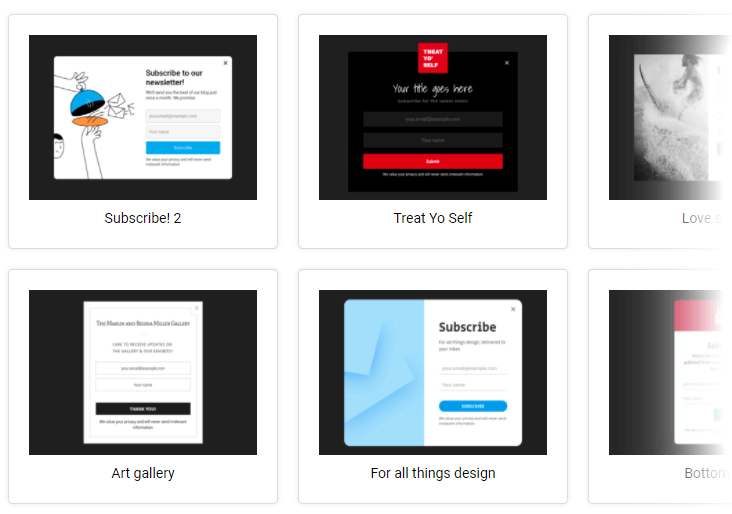This image is a screenshot featuring six distinct square templates designed to prompt users to subscribe to a website or newsletter. Each square contains unique text and visual elements, predominantly using a color palette of black, red, blue, and white. 

- The first square prominently displays the message "Subscribe to our newsletter" followed by the numerical code "85712."
- The second square features the text "Treat yourself" at the top and "Your title goes here" at the bottom, suggesting space for customizable content.
- The third square contains the phrase "Love something" and includes an image of someone surfing, adding a dynamic and adventurous visual element.
- The fourth square is labeled "Art Gallery," likely intended to appeal to those interested in visual and creative arts.
- The fifth square reads "For all things design," signaling a focus on design-related content.
- The sixth and final square simply states "Bottom," possibly indicating its position or placeholder text.

Together, these six templates offer various calls-to-action and visual styles to attract and engage website visitors or newsletter subscribers.